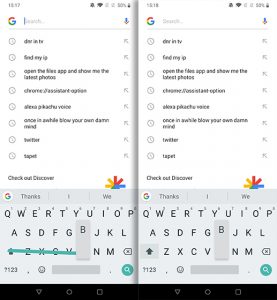This vertical rectangle image is composed of two cell phone screenshots placed side by side, creating one cohesive picture. Both snapshots are bordered by a black strip at the bottom containing three small, indistinct symbols. Moving upward from the bottom, each image features a grayish keyboard. The keyboard on the left has a strikethrough on certain keys, while both keyboards have a magnifying glass icon, signifying the search function, at the bottom right corner.

Above each keyboard, there is an emblem resembling a peacock. Following this, there's a list of items, each accompanied by an icon aligned on the left side. At the very top of each screenshot, there's the Google logo alongside search and microphone icons. The time is displayed on the upper left, although it is not clearly readable due to its small size. Finally, there are various status symbols, including Wi-Fi, a signal icon, battery, and battery percentage indicators.